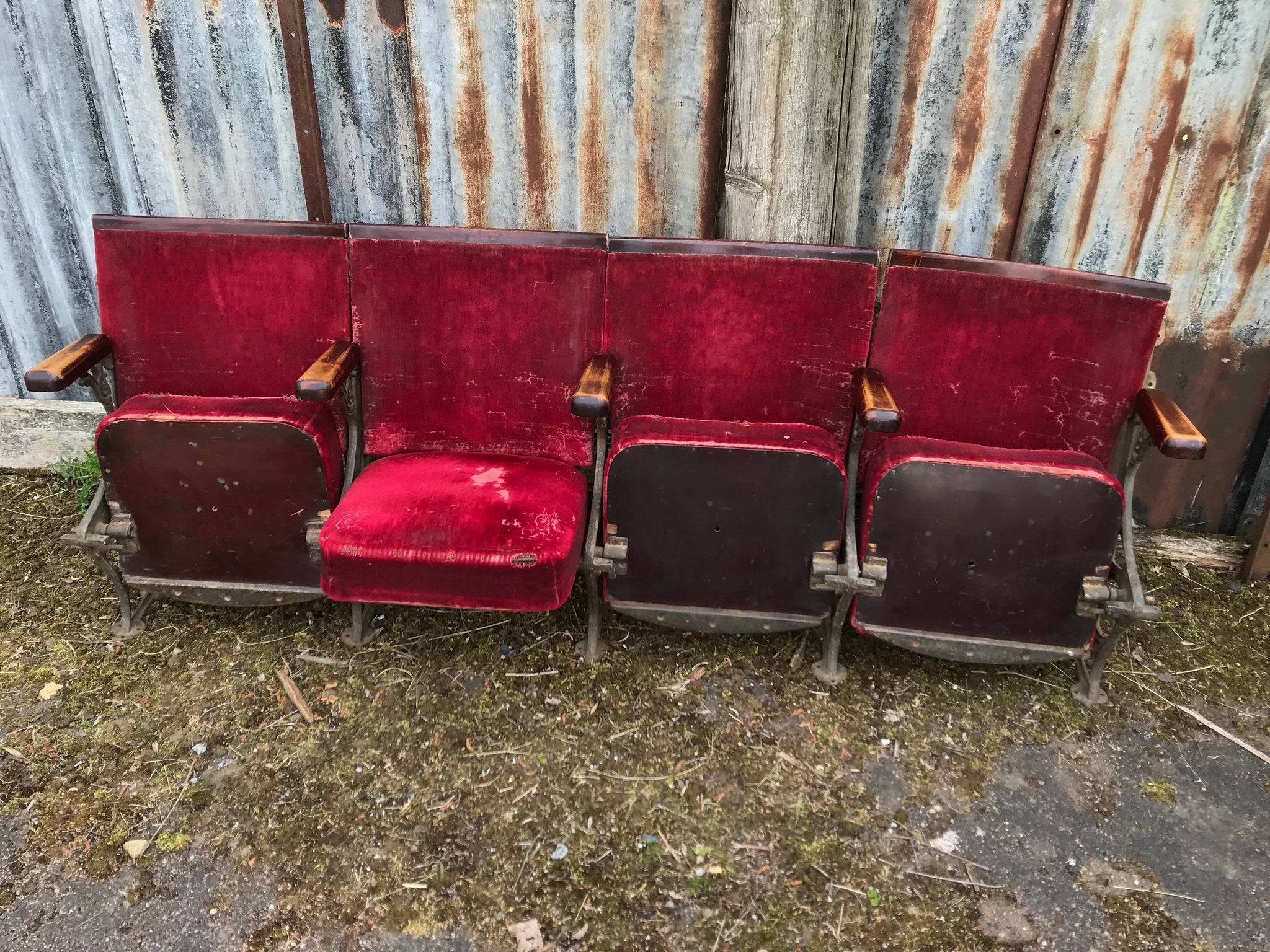The image showcases a neglected, outdoor scene featuring a row of four weathered, old-fashioned movie theater chairs. These chairs, upholstered in red velvet that's now faded and marred by scratches, are positioned against an aged, rusty fence that looks like a mix of old wood and corrugated iron. The chairs, which have seen better days, are set amidst patchy, scraggly grass with brown, dry patches of bare earth and some twigs scattered around. The seating arrangement shows variability in their condition: the first and the last two chairs have their seats folded up, while the second chair’s seat remains down, possibly due to a broken spring. The armrests of the chairs are short and dark in color, evidencing their age with noticeable wear. The entire scene suggests that these chairs have been discarded and left to the elements, with signs of bird excrement and rust adding to their deteriorated state.